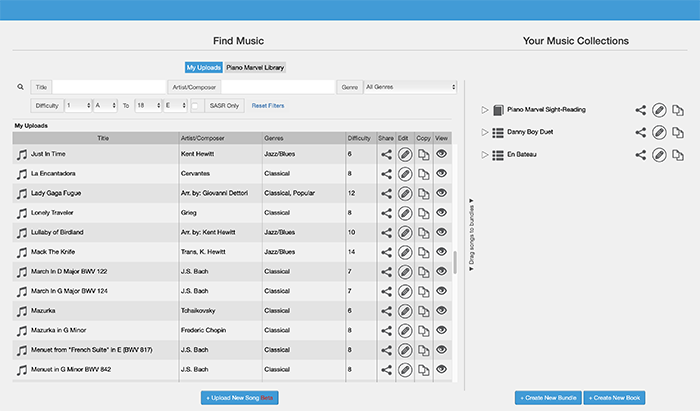A computer screen displays a music management interface with a light blue navigation bar at the top and a gray background. Beneath the bar, the heading "Find Music" is prominently displayed, followed by search options where users can input the title, artist, composer, genre, and difficulty level of the music they are looking for. To the right, a section titled "Your Music Collection" is visible. 

Below "Find Music," there are tabs labeled "My Uploads" and "Piano Marvel Library." The search options allow for filtering by all genres and various levels of difficulty. Under these search fields, a list of uploaded music is presented, detailing the title, artist and composer, genre, difficulty, and additional information about each piece.

Currently listed songs include "Just in Time" by Kent Howell in the jazz and blues genre, "La Somethin' Cervantes" in classical genre, and "Lady Gaga Fugue" by an indeterminate composer, also in the classical genre. The difficulty of these pieces ranges from 6 to 14, showcasing a wide variety of genres, with a particular emphasis on classical music.